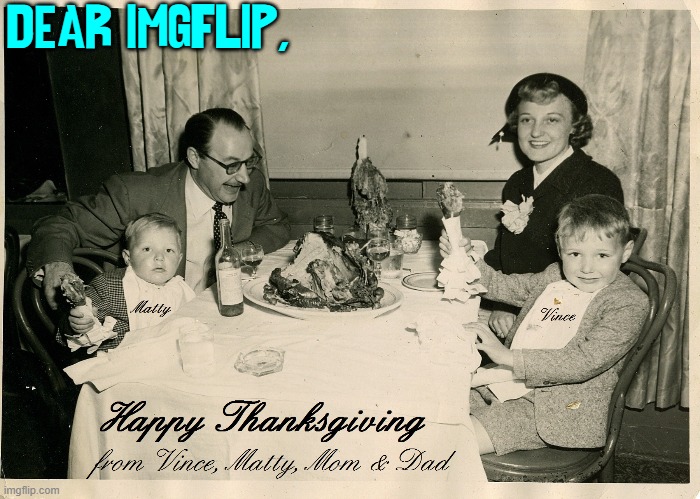This vintage black-and-white photograph captures a family of four enjoying their Thanksgiving dinner in a restaurant. The scene features a mother, father, and their two young boys seated around a dining table adorned with a white tablecloth. In the center of the table lies a thoroughly carved turkey on a platter, along with a candlestick with melted wax, a wine bottle, a clear ashtray, glassware half-filled with beverages, and various plates. The mother, positioned on the right, wears a black blazer with a corsage and a hat with a feather, smiling warmly. Next to her, Vince, the fair-haired boy, is also smiling, holding a turkey wing and wearing a blazer with a bib displaying his name. On the left side of the table sits the father, bespectacled and with receding hair, sporting a suit with a polka dot tie and grinning broadly. Beside him is the other son, Maddie, also light-skinned and fair-haired, wearing a suit jacket, shorts, and a bib with his name, holding the other turkey leg. The backdrop includes curtains and what seems to be a whiskey bottle. The bottom of the photograph is inscribed in cursive with, "Happy Thanksgiving from Vince, Maddie, Mom, and Dad," and the top corner bears the turquoise text, "Dear IMG Flip, comma."